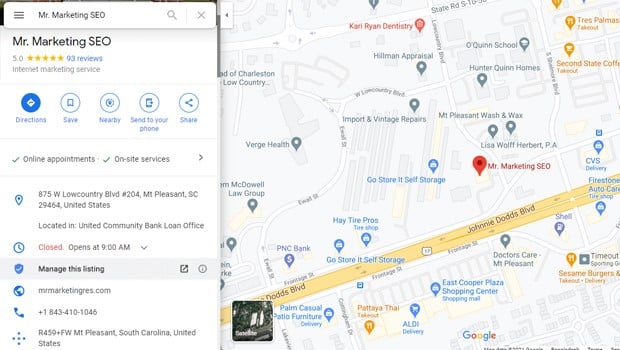The image features a detailed online map layout. In the upper left-hand corner, there is a hamburger icon represented by three horizontal lines. Next to this icon, the text "Mr. Marketing SEO" is displayed. Adjacent to the text on the right side, there is a search bar with a magnifying glass icon, accompanied by a separation line and an 'X' icon within the search bar area, forming a rectangular box.

Below this, the name "Mr. Marketing SEO" appears again in bold with a five-star rating and 93 reviews indicated underneath. Smaller informational text is present beneath the reviews. 

Subsequently, there are five icons, with "Directions" prominently highlighted. Next to it are options such as "Save" and a few others which are blurred out.

A thin line separates this section from the next, which lists services: "Online Appointments" and "On-Site Services," both checked. A right-pointing arrow is also displayed here.

Further down, the location information is listed comprehensively:
- Address: 875 W. Lowe County Boulevard, No. 204, Mount Pleasant, SC 29464, United States.
- Hours of operation state: "Closed, opens at 9 a.m."
Below this section, links to manage the listing, the website, and the phone number are provided, followed by additional directions at the bottom.